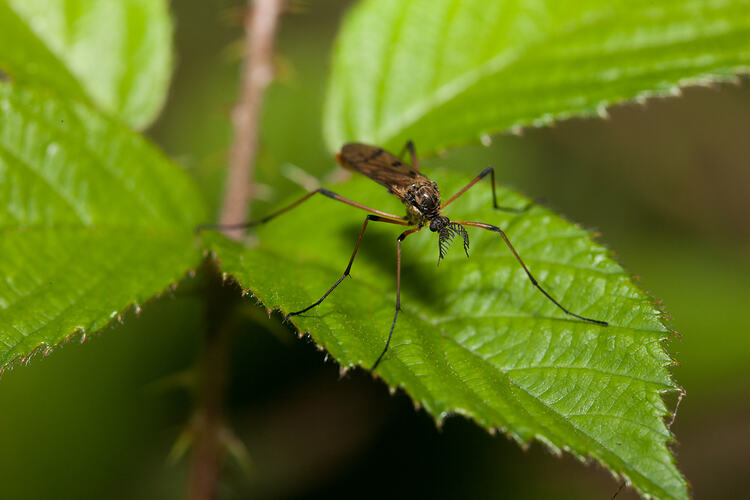This photograph captures an exceptionally detailed, close-up shot of an insect, potentially a mosquito, resting on a pristine green leaf. The insect, characterized by its brown color, slender, long legs, and translucent wings, sits centrally in the image, which is sharply focused on its minute features, including its small, black face. The leaf it perches on appears flawless, devoid of any imperfections or dirt, enhancing the sense of an almost surreal, pristine natural setting.

The framing of the image includes several other leaves and a pinkish-brown vine, which enter the frame from various angles. However, these surrounding elements are out of focus, creating a soft, colorful blur that draws the viewer's attention directly to the insect and its immediate green leaf perch. The background primarily showcases various shades of green, adding to the natural ambiance of the scene. The overall composition of the image emphasizes the intricate details of the insect while the peripheral blur accentuates its central prominence.